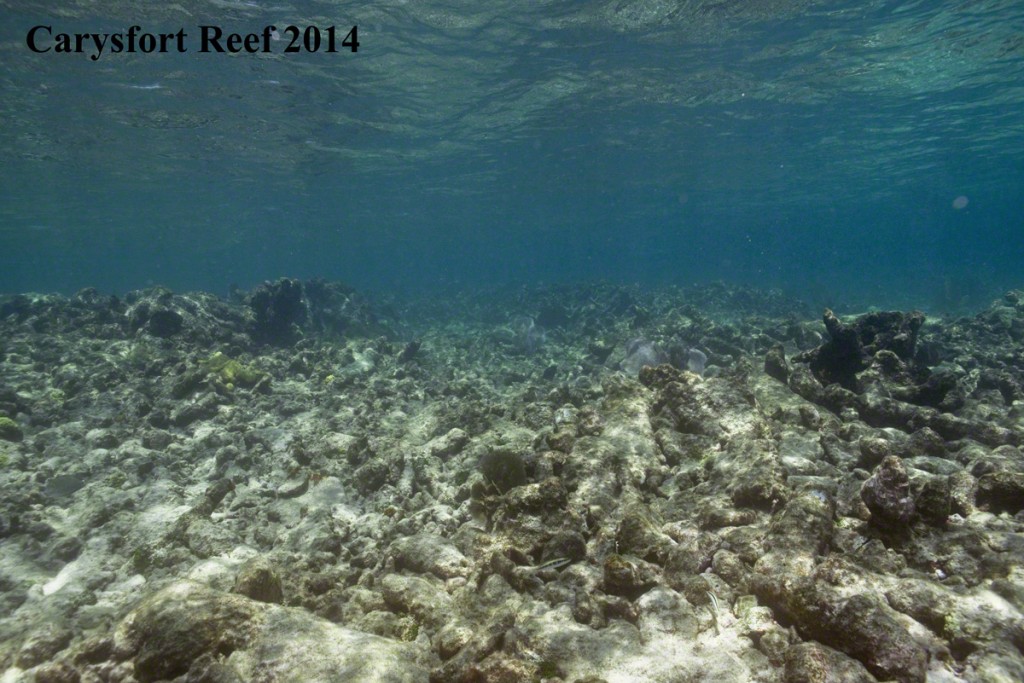The underwater photograph captures the stark reality of the Carries Fort Reef in 2014, as indicated by the text in the upper left corner. The top half of the image reveals a bright, sunny day with sunlight piercing through 20 feet of shallow, muted grayish-blue water. The bottom half showcases the damaged reef system, which is predominantly a mix of bleached white, gray, and dark mossy green corals, interspersed with splotchy white areas. The once-vibrant reef appears lifeless and diseased, devoid of fish and lush vegetation, resting on an ocean floor composed of variously shaped rocks ranging from white to brown. The overall scene is somber, highlighting the dramatic contrast between the brilliant surface light and the desolate underwater landscape.